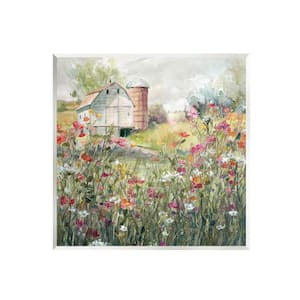This image depicts a small square painting, possibly watercolor, reminiscent of a greeting card. The scene features a bright, impressionistic meadow filled with an array of wildflowers including oranges, pinks, yellows, whites, and reds, set against a backdrop of vibrant green grass. Some of the flower stalks have a bluish-green hue. The meadow leads to an older white barn, which stands upon a platform and is topped with a rust-colored roof and a weathervane. Next to the barn is a brown silo with a rounded silvery-gray metal roof. Further back, a hillside can be seen on the left, adding depth to the landscape. The background is comprised of impressionistic trees and a sky filled with gray and pale white clouds, giving the scene a tranquil yet slightly somber atmosphere. The painting is detailed with elements that draw the eye towards the bright flowers in the foreground, contrasting beautifully with the muted colors of the sky and the rustic architecture of the barn and silo. A thin white border frames the painting, emphasizing its small, intricate craftsmanship.